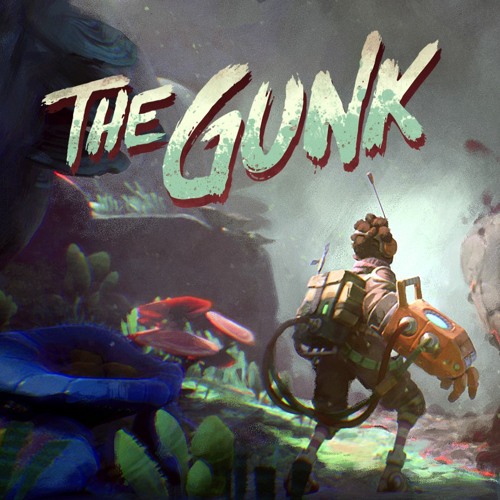In this detailed, digitally created image, a man is featured standing on the ocean floor, wearing a full scuba gear tank on his back. He is positioned in a square format illustration, facing towards the right, and his stance is a mix of standing and slightly crouching. He dons shorts, a beige shirt, and sophisticated equipment, including a bulky metal apparatus on his right hand that's connected via cables to his backpack. This apparatus is orange with a clear window on top and serves as a significant visual cue, adorned with an antenna.

The setting is a fantastical underwater scene with rich details, including flowers, grass, and various marine structures. Notably, there’s a prominent rocky formation and blue and red mushroom-shaped objects at the bottom left corner. These elements enhance the vibrant background, filled with mint green, beige, orange, red, blue, dark green, light green, and off-white hues.

At the top of the image, against the ethereal background, there's a bold brushstroke heading that reads "THE GUNK." This text has a speckled treatment, transitioning from cream to light green. The overall style of the illustration combines 3D fantasy with graphic design elements, creating a visually striking and imaginative underwater scene.